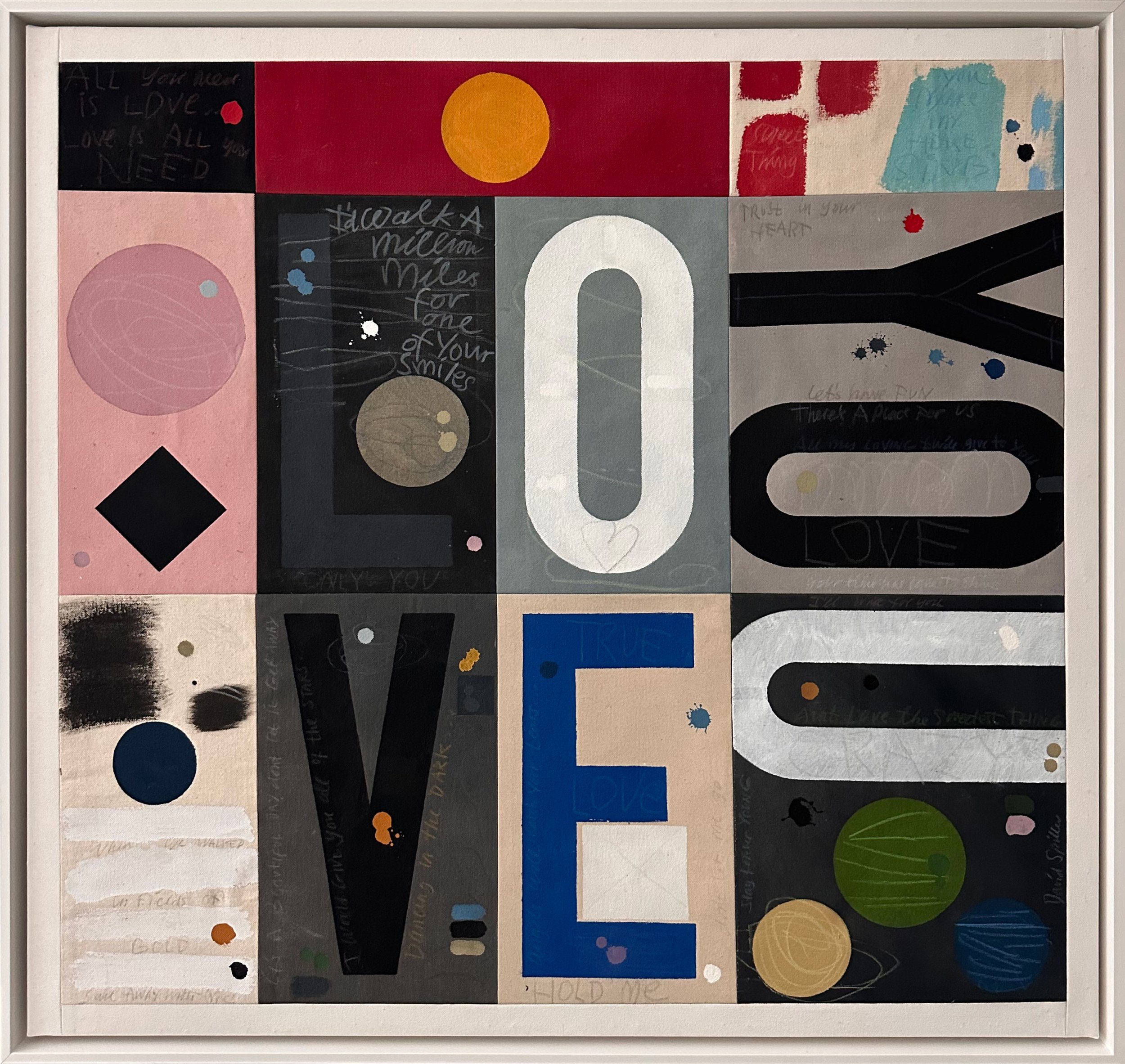A contemporary artwork in a minimalist white frame featuring a collage of diverse panels, each uniquely colored and adorned with various objects and letters. The composition is thoughtfully arranged in a grid pattern. The first panel is a stark black background with a striking red dot. Adjacent to it is a red space highlighted by a yellow dot. Another panel showcases a beige background with random splatters of red and blue paint, creating a dynamic visual texture. A contrasting pink panel features a pink circle alongside a black diamond shape. Additional panels include white rectangles with the letter "O," the word "YOYO" in bold black letters, and a combination of letters – L on a grayscale background, V in black, and E in blue – collectively spelling out the phrase "LOVE YOU," although an "I" appears to be absent from the composition. Each element contributes to the overall abstract and eclectic aesthetic of the piece.